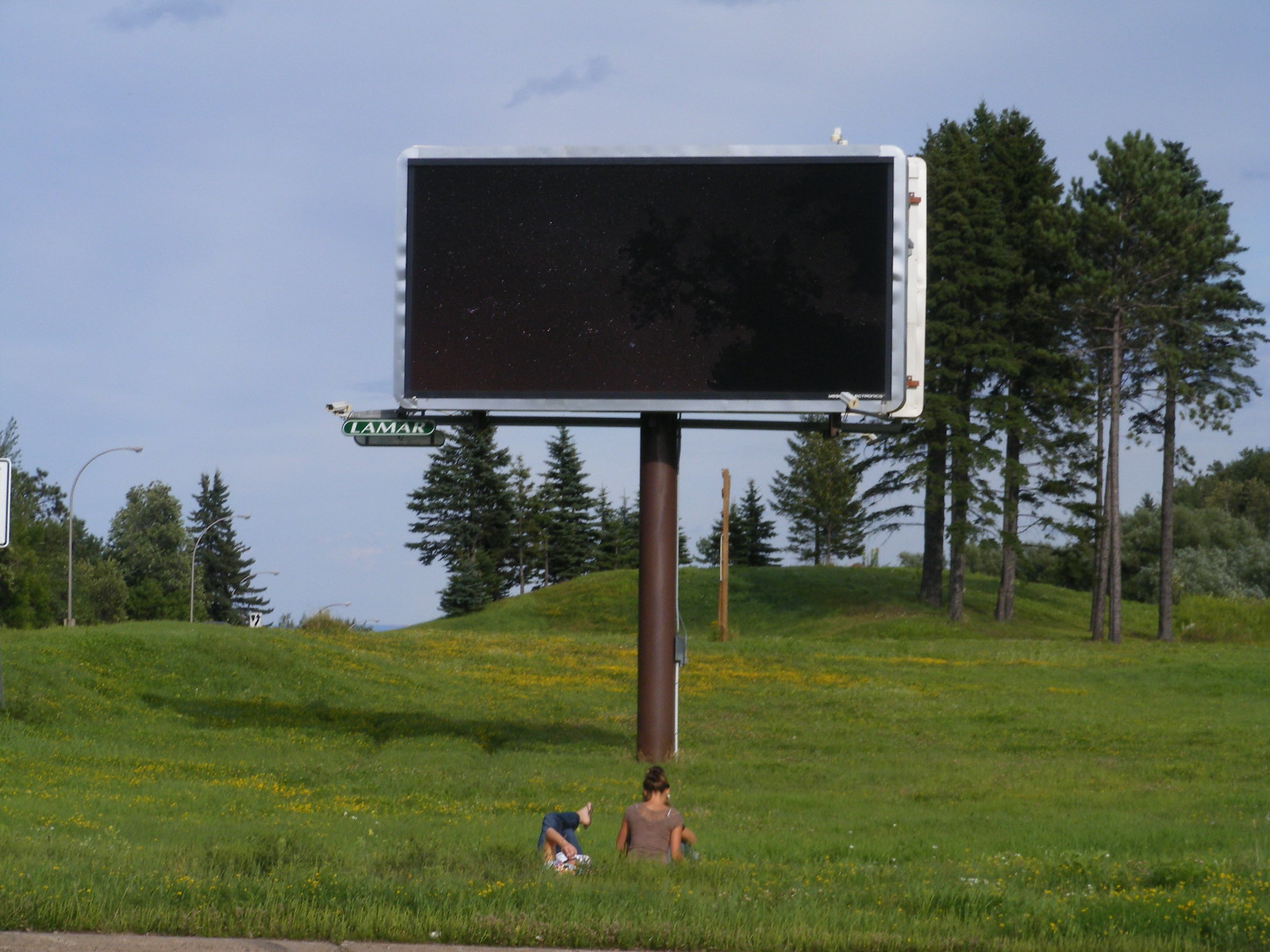The photograph captures a bright, sunshiny day in a picturesque landscape reminiscent of "Teletubbyland," featuring a grassy meadow with gentle mounds and hills. A distinctively jarring digital billboard, elevated by a tree trunk-like brown pole, dominates the scene's center. The billboard, currently blank with a black screen and bearing the name "Lamar," stands in stark contrast to the natural beauty surrounding it. Two people are in the foreground: a woman with dark hair, styled in a bun, who is sitting up on the grass possibly making a daisy chain, and another person lying down with legs crossed over the woman’s lap, both surrounded by yellow poppies. In the distance, the meadow slopes towards a highway, explaining the presence of the billboard, and is bordered by a variety of lush, green trees. A couple of streetlights are visible far off, punctuating the serene, rolling landscape under a light blue sky.